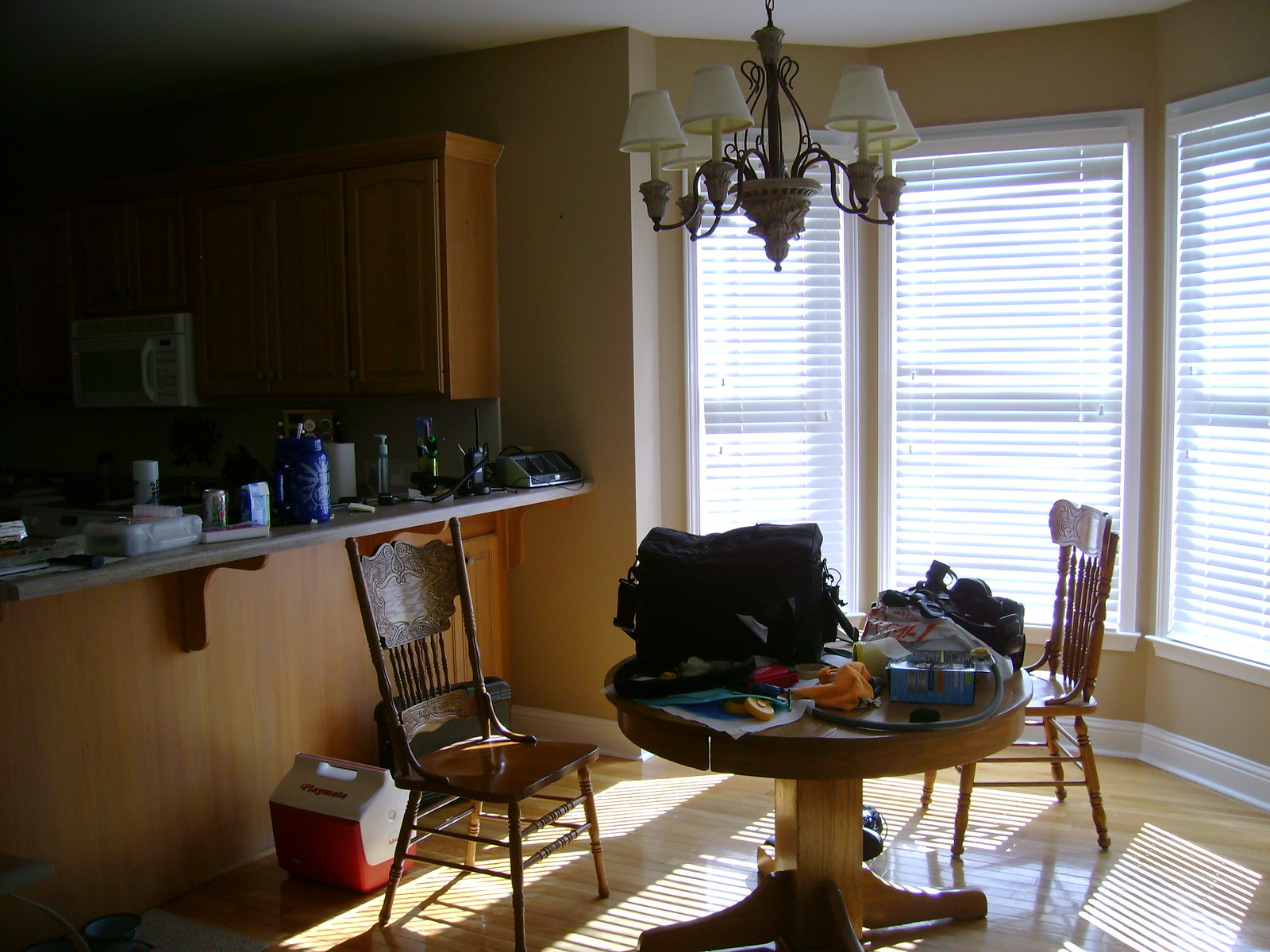The dining area, bathed in natural sunlight filtering through the window blinds, exudes a warm and inviting ambiance despite the absence of artificial lighting. Three windows framed in pristine white with matching lintels allow the daylight to flood the space, enhancing the elegant beige walls in a very light shade of brown. The polished hardwood floor in a pine hue adds a cozy and homely touch. The centerpiece of the room is a robust wooden dining table featuring a solid block stand with a four-legged base. Surrounding the table are chairs crafted from shiny, polished deep brown wood, reflecting meticulous craftsmanship. Atop the table, a black bag and several miscellaneous items are scattered. Overhead, a chandelier with mini lamps encircles its frame, adding a touch of sophistication and charm to the room.